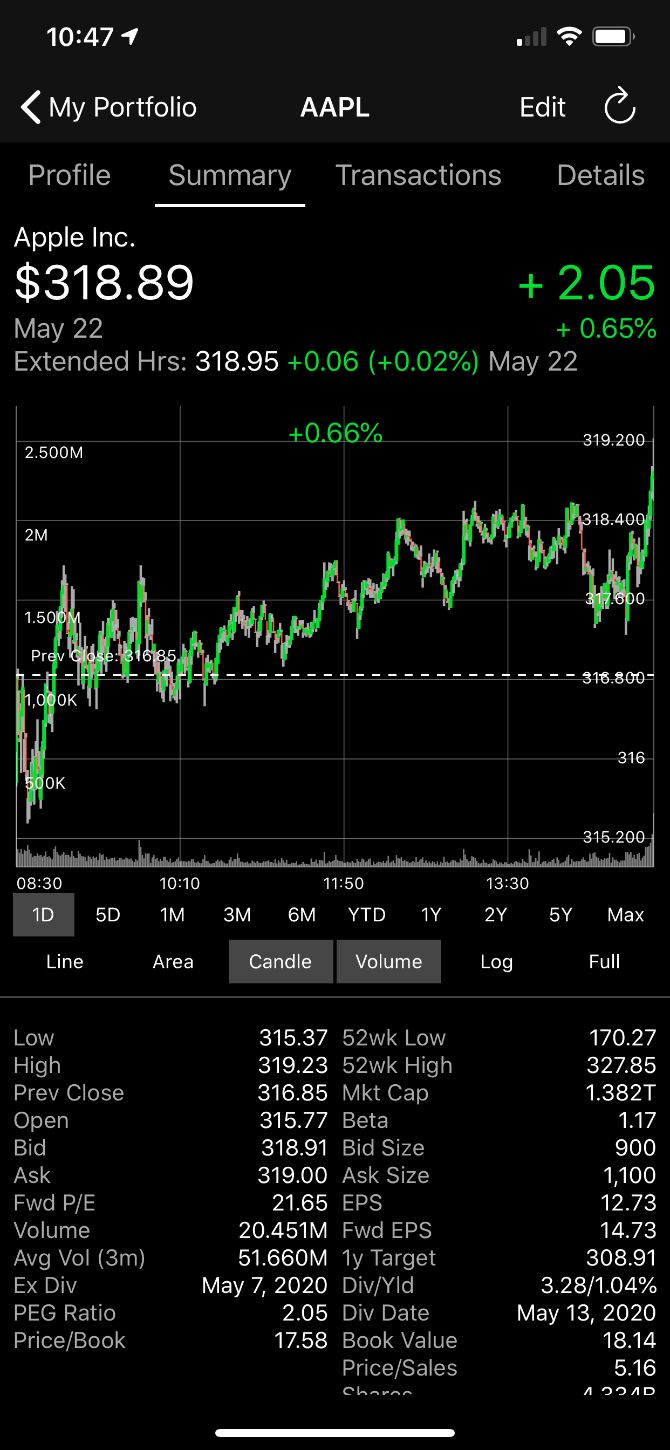The image features a detailed financial dashboard with a sleek, professional design. Dominating the top section is a long black box with a timestamp of "10:47" on the left, and to the right, a horizontal white battery icon indicating power status.

Below that, the content begins with an arrow pointing left, followed by the text "My Portfolio." Centrally placed and prominently displayed is "AAPL" in all capital letters, signifying Apple Inc.'s stock symbol. To the right of this, the word "Edit" appears next to an arrow pointing right, suggesting customization options.

Beneath this header section, there is a navigation bar with options labeled: "Profile," "Summary" (which is underlined indicating it is the current selection), "Transactions," and "Details."

Further down, the stock details for Apple Inc. are shown. "Apple Inc." is followed by a period, with the current stock price listed as "$318.89." Below this, the extended hours price is "$318.95," with a green increment of "+0.06" dollars enclosed in parentheses along with "+0.02%." The date "May 22nd" is also displayed.

On the right above the stock price, formatted in smaller green text, is a change of "+2.05" points followed by a smaller percentage increase of "+0.65%." Continuing downwards is another percentage figure, "-0.66%," possibly referring to a different time frame or comparison metric.

Centrally placed is a stock price graph illustrated with green lines displaying erratic upward and downward movements, signifying a volatile trading period with no easily discernible pattern.

Finally, below the graph, two gray boxes are positioned with the labels "Candle" and "Volume," likely offering different ways to view the stock data.